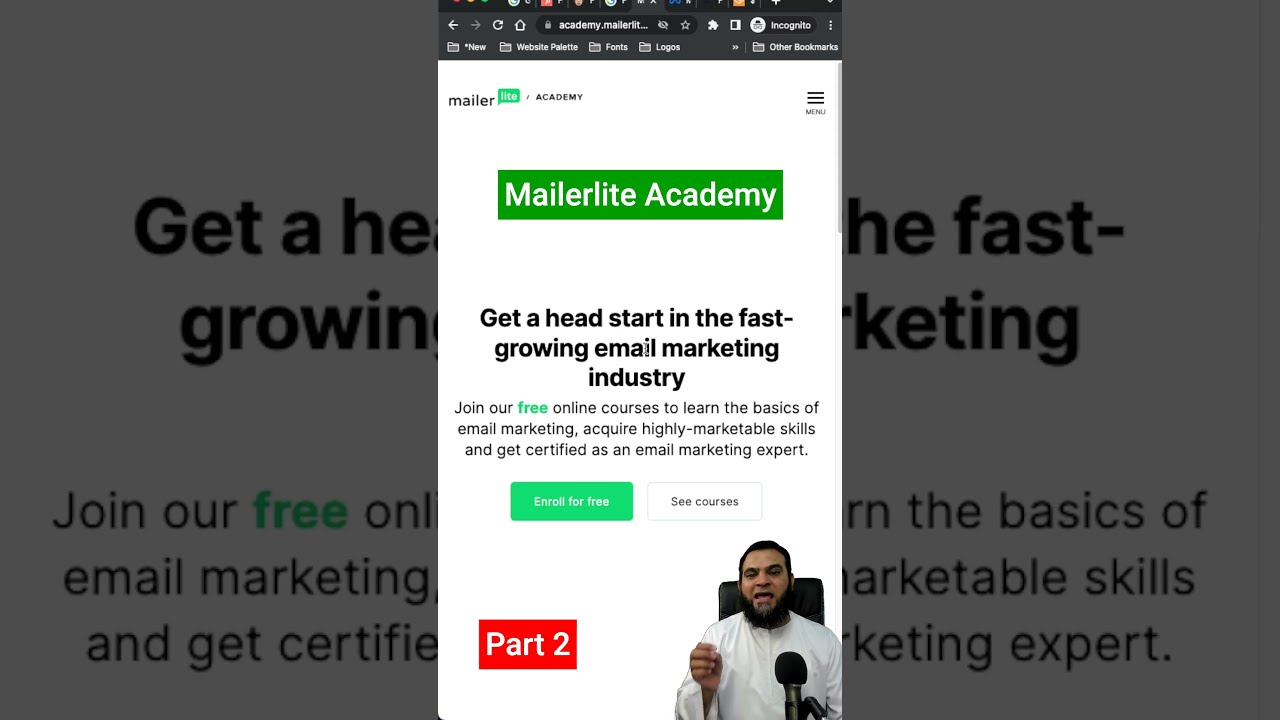The image is a horizontal rectangular screen capture from a cell phone, featuring an advertisement for Mailer Light Academy. At the top is a browser interface with icons like home, refresh, and navigation arrows, along with an address bar. In the center of the image, the ad consists of several elements on a grayed-out background resembling an article related to the ad content. 

The ad prominently displays a green rectangular box at the top with the text "Mailer Light Academy" in white. Below this, in large black text, it reads, "Get a head start in the fast-growing email marketing industry." This message is followed by a description in smaller black text: "Join our free online courses to learn the basics of email marketing, acquire highly marketable skills, and get certified as an email marketing expert." Below this description, there are two green buttons labeled "Enroll for Free" and "See Courses."

At the bottom of the ad, a red rectangle with white text reads "Part 2." Towards the bottom right corner of the image, there's a picture of a man with short dark hair and a full beard, wearing a white shirt or robe and sitting in a high-backed black chair. He is speaking into a microphone and gesturing with one hand, indicating he might be giving lessons for the Mailer Light Academy.